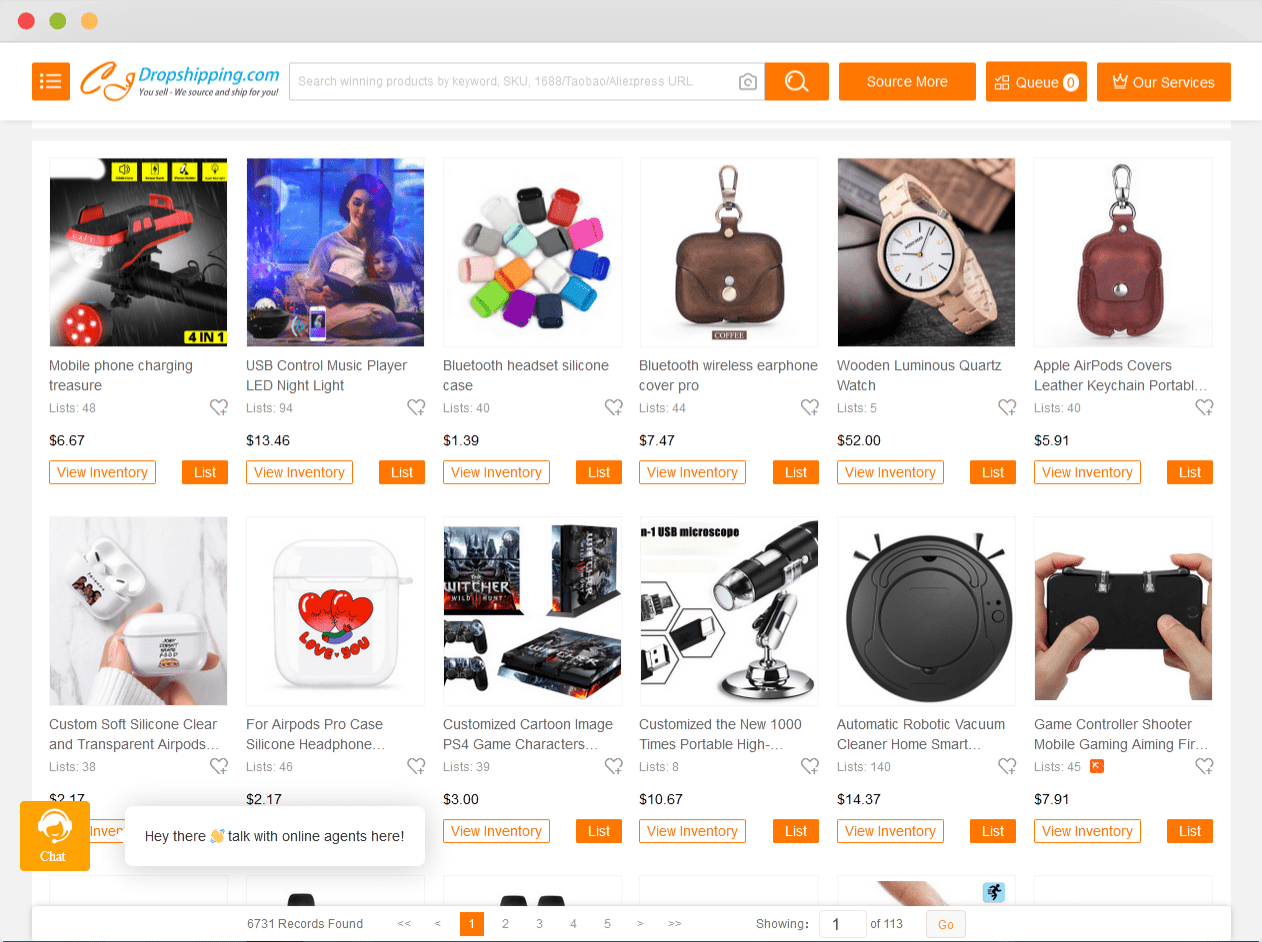The image comprises a series of colorful squares, each detailing different products and services. Starting at the top, a red square features the text “dropshipping.com” alongside the instruction to "search for an appropriate keyword." Adjacent to it, an orange square mentions "Metronauts," advising users to "search for QR services."

Below, a grid of product listings begins:

1. A square highlighting "Mobile Phone Charging" with reference number 48, 6167, leading to an inventory view.
2. Next, a "USB Control Music Player" paired with an LED nightlight, listed under 1346, with an inventory view option.
3. A "Bluetooth Headset" and "Silicone Case" with its listing number 44, 747, leading to inventory details.
4. Following that, a "Bluetooth Wireless Earphone Cover Pro" is mentioned, listed similarly under 44, 747.
5. A "Wooden Luminous Quartz Watch," described as resembling a traditional school watch, priced at $52, includes a link to its inventory.
6. "Apple AirPods Covers," which feature leather keychains and are red, are marked with list number 45, 91.
7. Custom "Soft Silicone Clear and Transfer AirPods" cases, designed for AirPods Pro, feature customized carbon images and PS4 game characters.
8. A "Neo 1000 Times Portable High Precision Automatic Robotic Vacuum Cleaner" for smart homes, mentioned under number 1437.
9. A "Game Controller Shooter" designed for mobile gaming, particularly for aiming purposes.

The scene concludes with a mention of numerous agents, five in total, who are presumably involved in managing the products and services displayed.